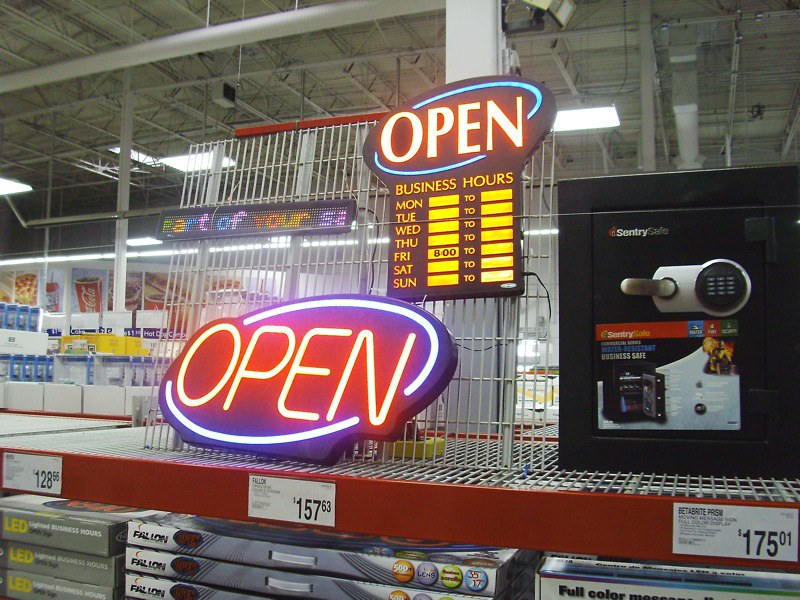The image captures a display inside a store showcasing various items and signs available for purchase. A prominent feature on the right side is a black safe adorned with decorative stickers in yellow and white, displaying a circular, numbered lock and priced at $175.01. Adjacent to the safe, there are two glowing "Open" signs. The first "Open" sign in red with blue outer linings is priced at $157.63. Positioned above this, another "Open" sign includes a section indicating business hours, with days of the week listed on the right and specific hours underneath; notably, Friday's hours read 8-2. The shelves, supported by red beams and metal wire racks, also display other items such as what appears to be a long rectangular LED sign with changeable lettering. Price tags for various items range from $128 to $175. In the background, parts of a Coca-Cola sign and another digital display reading "part of your" can be seen, contributing to the store's eclectic assortment of products.